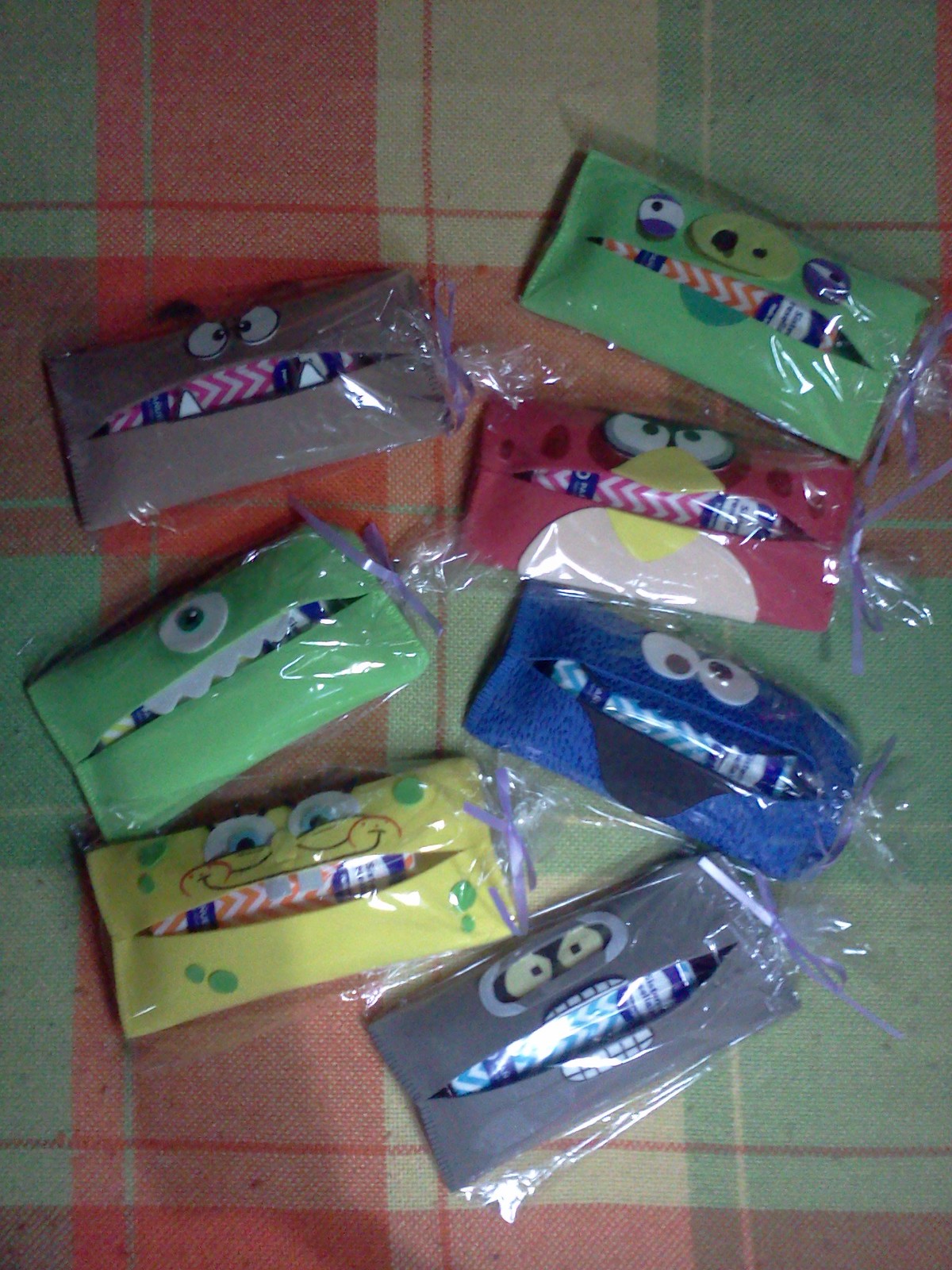This is a detailed color photograph displaying seven rectangular, clear plastic-wrapped containers designed for kids, resembling characters from popular TV shows and games. The containers are arranged on a tartan fabric tablecloth with red, green, and beige checks. Each container has a slit in the middle, designed to resemble a mouth, ideal for dispensing items like tissues. The plastic wrapping is secured with lavender-colored ribbons. From left to right, top to bottom, the characters depicted include a Goomba from Mario, Mike Wazowski from Monsters, Inc., Spongebob Squarepants, a pig from Angry Birds, an Angry Bird, Cookie Monster, and Bender from Futurama. Each character container is adorned with playful, exaggerated facial features, making them look fun and engaging for children.